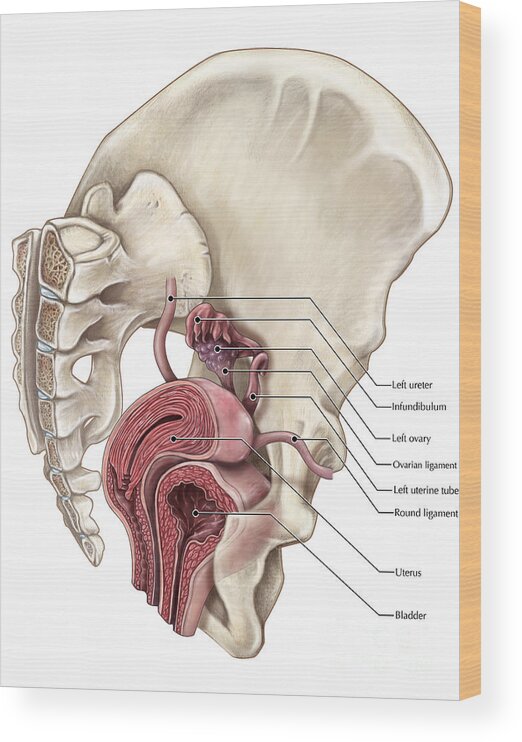This detailed anatomical drawing on the canvas focuses on a cross-section of the female reproductive system and surrounding structures. Prominently displayed is the left side of the pelvis, with a large hip bone and segments of the spine visible on the left-hand side. The illustration features meticulous labeling of various reproductive organs: the left ovary, ovarian ligament, left uterine tube, round ligament, uterus, left ureter, and bladder. The depiction is complemented by a series of approximately ten call-outs with black arrows identifying these key elements. The image juxtaposes reproductive and some urinary anatomy, highlighting the intricate relationships between these systems. Additionally, layered muscle sections, varying in thickness and depth, are shown, providing a comprehensive view of the internal anatomical structure. The drawing serves as an educational guide, emphasizing the interaction between the skeletal and reproductive systems.